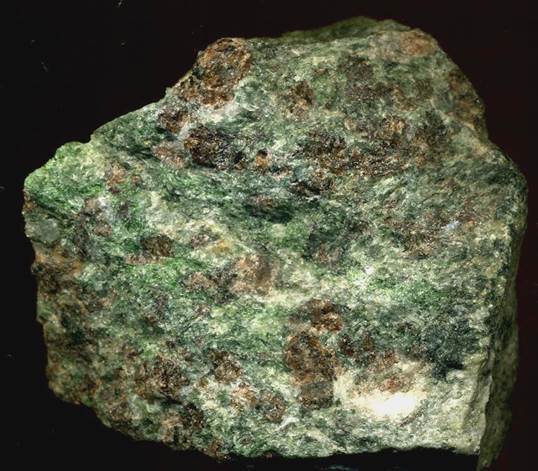The image showcases a large, unpolished, pyramidal-shaped rock set against a completely black background, implying an indoor setting. The rock, which dominates the frame, is primarily emerald green with varying shades and earthy tones visible throughout its rough, textured surface. There's an intricate interplay of colors with noticeable splotches of white and sporadic dark brown or blackish marks that resemble burn marks. The rock's outline is characterized by a diagonal ascent from the left, followed by a steep incline toward the middle and a downward slope to the right. The light source illuminates one side of the rock, revealing its rugged details and creating a striking contrast with the deep black backdrop.